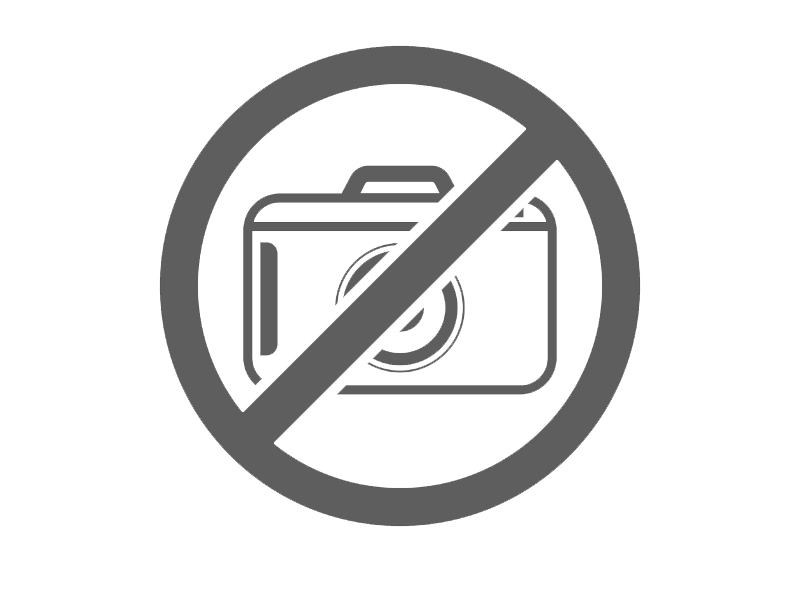This image is a high-quality PNG computer graphic designed as a clear and simple warning label indicating "No Photography" or "No Cameras Allowed." The graphic is set against a translucent or white background and measures approximately four inches by four inches. It features a medium gray circular design with a diagonal line running from the upper right to the bottom left, symbolizing prohibition. At the center of the circle is an outlined image of a camera, depicted in a simplified, line-art style. The camera is a basic rectangular shape with rounded corners, a circular lens in the middle, and a small protrusion at the top representing the flash or a button. The entire design is minimalistic, devoid of intricate details or text, serving effectively as a universal pictogram to communicate the restriction visually and without language barriers.